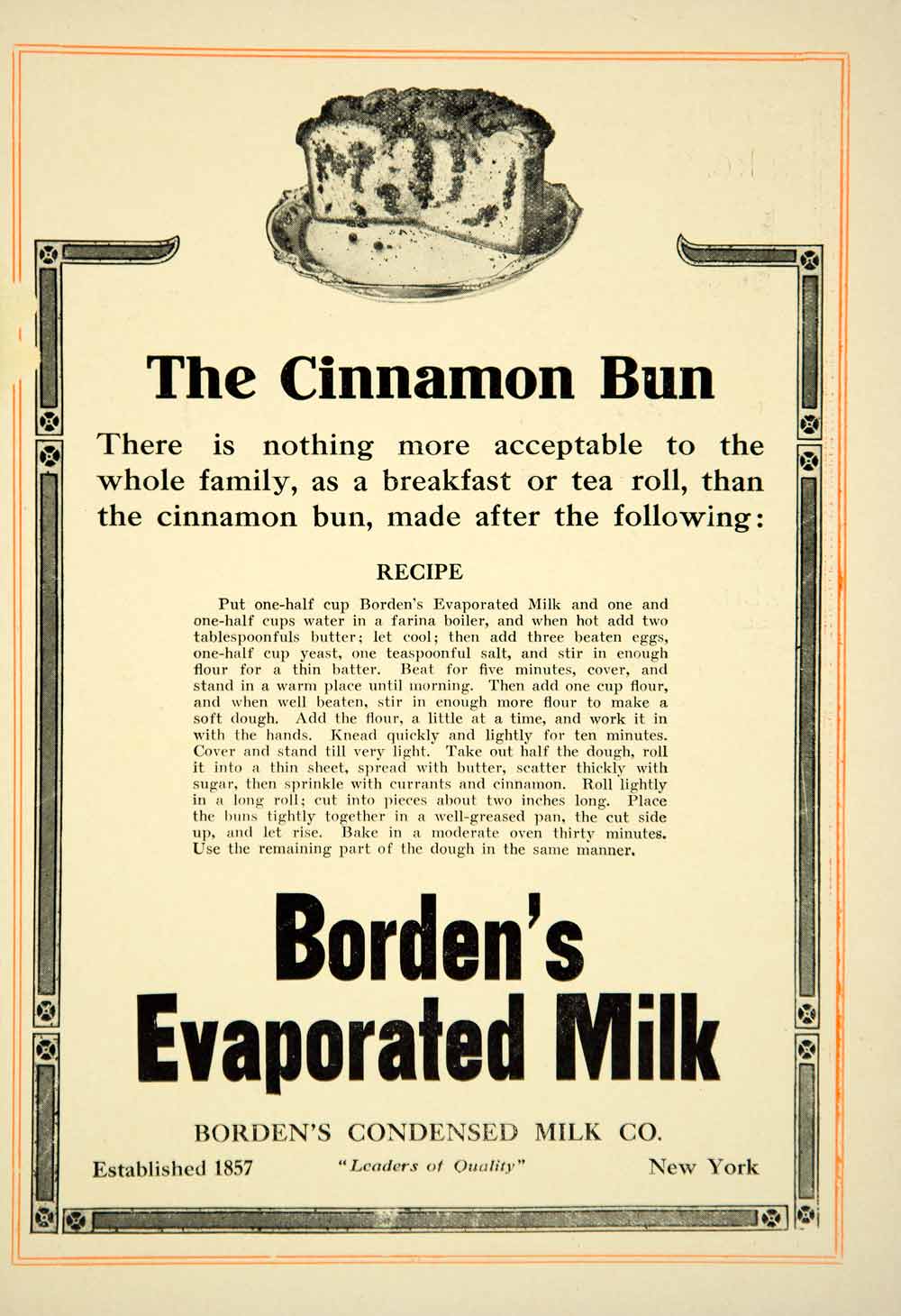This vintage-style poster, set against a light brown background, prominently features the title "The Cinnamon Bun" at the top. The header is accompanied by a detailed black-and-white drawing of a cinnamon bun, cut in half and displayed on a plate. Below the illustration, the text reads: "There is nothing more acceptable to the whole family as a breakfast or tea roll than the cinnamon bun, made after the following recipe." This statement is followed by a long paragraph of text presenting the recipe, printed in a smaller, more challenging-to-read font. At the bottom, in larger letters, it announces: "Borden's Evaporated Milk, Borden's Condensed Milk Co. Published 1857, Leaders of Quality, New York." The entire text is framed with a black border, which is again surrounded by a larger orange border, emphasizing the classic and historic aesthetic of the advertisement.